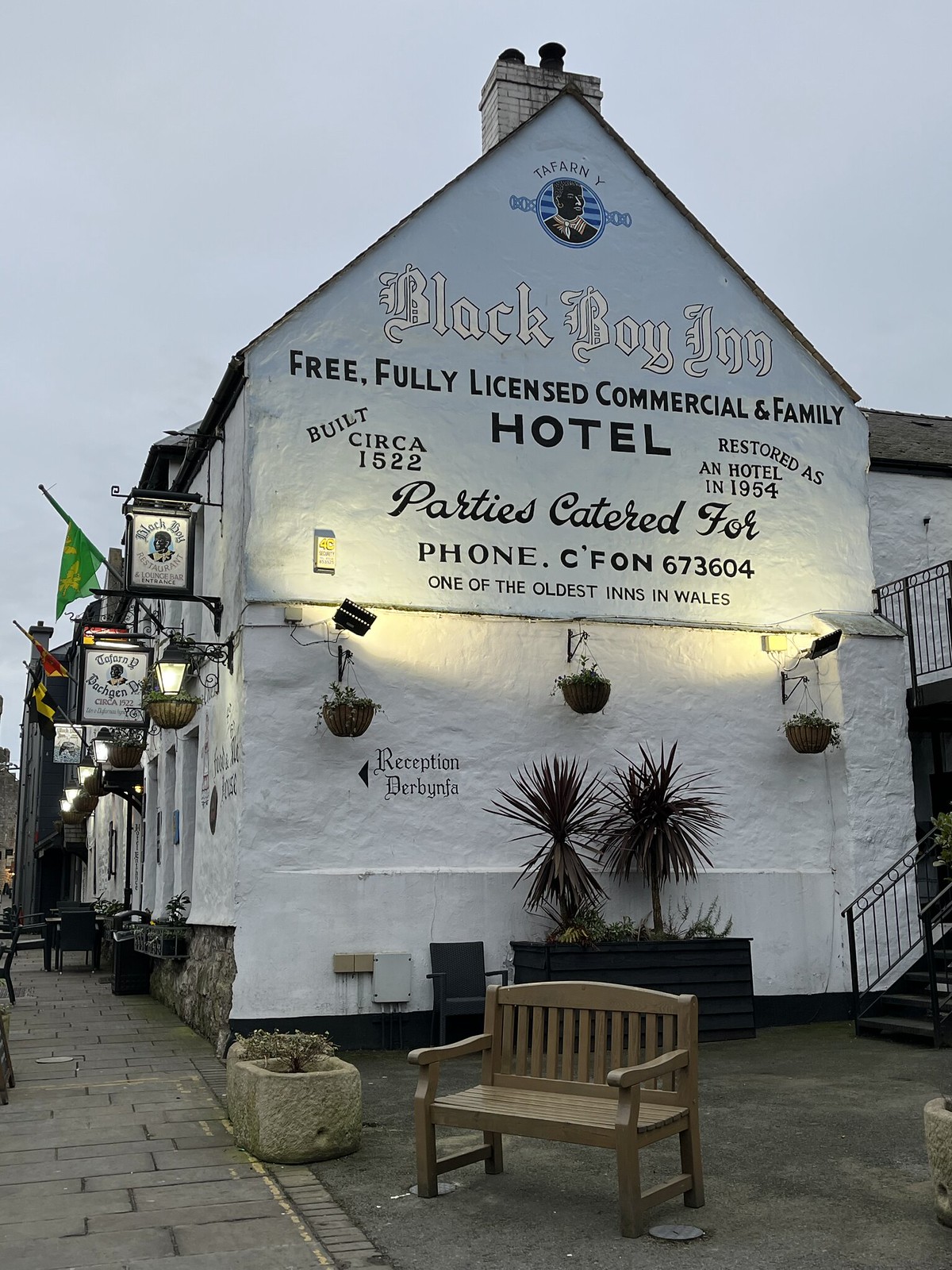The photograph captures a quaint scene at dusk or just after sunset, highlighting a historical two-story building made of painted white stone. The sky above features a shadowy blue hue, indicating the waning light of early evening. The signage on the side of the building prominently displays the text: "TAFARN-Y Black Boy Inn. Free, Fully Licensed, Commercial and Family Hotel. Built circa 1522. Restored as a Hotel in 1954. Parties Catered. Phone 673-604," along with "Reception" and an arrow pointing toward the front of the building. The building also features an intricate wrought iron design, including framed signs and hanging flower baskets. It is adorned with potted plants and stone planters around its base. An ornate chimney crowns the triangular roof of this edifice, bearing the logo of a man's face within a circle. There is an elaborate brick sidewalk and a wrought iron staircase leading up to the right side of the building. Lights illuminate the various signs, and nearby, a wooden bench invites passersby to sit. This picturesque spot is part of a charming and historically rich neighborhood in Wales, offering a glimpse into its storied past.